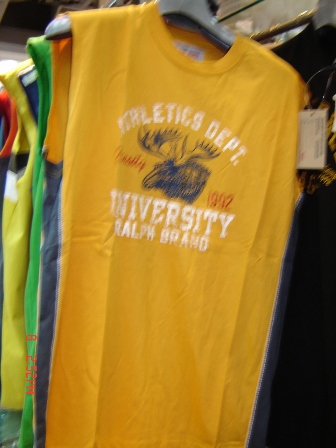In this image, there is a standalone rack of sleeveless shirts, reminiscent of jerseys, displayed at what appears to be a department or clothing store. The shirts come in a variety of vibrant colors, including shades of yellow with blue trim, green with black and white trim, and more. Each shirt is neatly hung on a white hanger and features tags. The design on the shirts includes the words "Athletics Department" in white at the top, "1992" in the middle alongside an image of a moose, and "University Ralph Brand" at the bottom. The rack itself seems to be positioned independently, with no other items surrounding it, indicating that this is likely the front of the display.